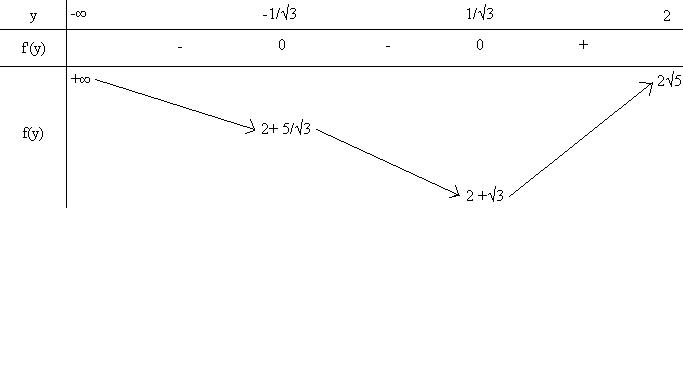This image depicts a detailed mathematical grid focusing on an equation involving both the X and Y axes oriented downwards. The grid is divided clearly and structured in a systematic manner. In the top left corner, there is the variable 'Y,' which is separated by a horizontal line from the column below it. Directly underneath this 'Y' in the next cell is the notation 'f(Y)' followed by another 'f' below it in the next cell down, forming a vertical sequence in the same column. 

To the right of the initial 'Y' symbol, various mathematical notations are spread out. These notations include the symbols for infinity (∞) and negative infinity (-∞), with the latter slightly above and to the right of the former. Further to the right of these symbols can be seen numbers and mathematical constants including -1, √3 (square root of 3), and positive 1. These continue up to a value of 2 in ascending order.

On a lower horizontal line below the initial set of numbers, there are zeros aligned under respective numbers. These zeros are separated by minus (-) and plus (+) signs, indicating different mathematical operations. Below this arrangement, the notation 'plus ∞' appears in the top left of the blank space, signaling a transition in the calculations.

From this point, a diagonal arrow points downwards to the right, leading to the expression '2 + (5/√3).' Following this expression, another downward arrow points to '2 + √3,' and an arrow further leads to the notation '√5,' connecting the series of calculations. 

Overall, the image visually represents a step-by-step mathematical sequence detailed with various equations and notations, structured within a clearly defined grid.